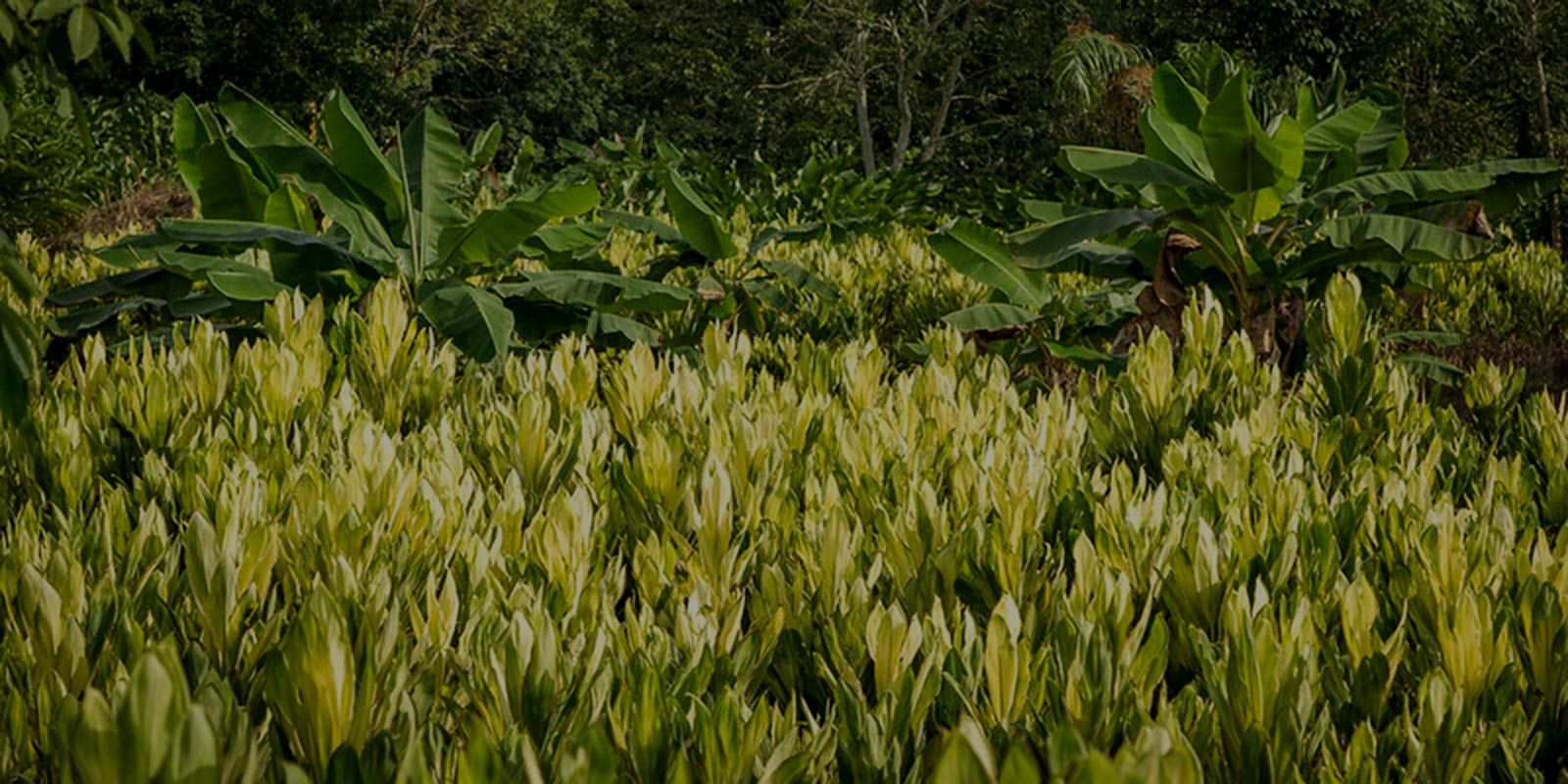This photo captures a vibrant and dense field of crops or tropical plants that creates a rich, layered tapestry of green hues. In the detailed foreground, light green, pointy leaves with hints of yellow are tightly clustered together, forming bunched colonies that exude a vigorous growth. Gradually leading your eyes further into the scene, two distinctive clumps of darker green plants, possibly young palm or banana trees, stand taller amidst the lighter vegetation. Their wide, dark green leaves create a recurring pattern that extends towards the horizon, enhancing the impression of a meticulously spaced farm plantation. In the distant background, a densely wooded area with darker green trees and bushes adds depth and contrast to the image. The rich greenery gradually darkens, merging into a dense forest that suggests a thriving plantation nestled in the heart of a wild, natural setting.